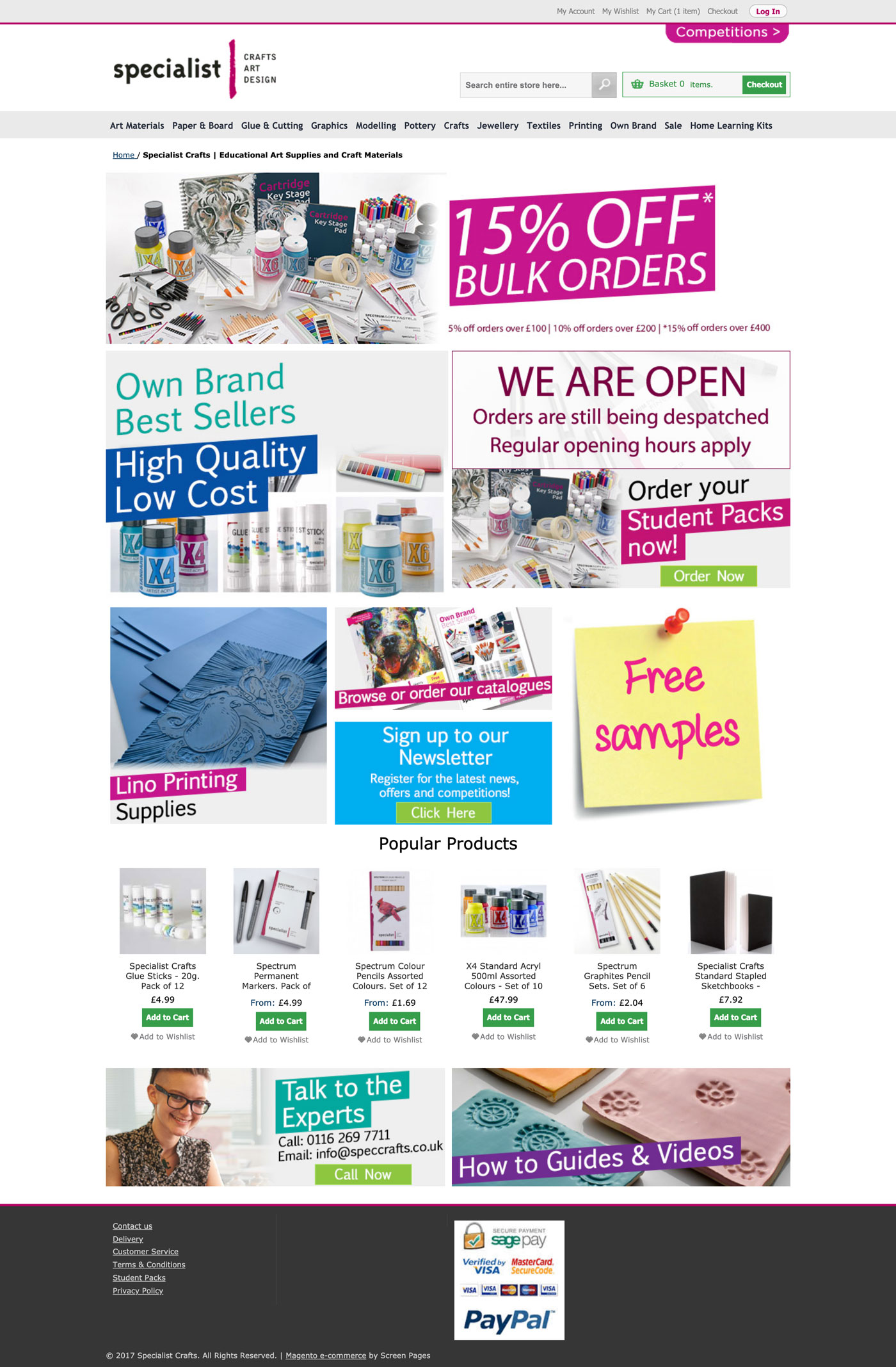This image captures a screenshot of a British website called "Specialist" that focuses on Crafts, Art, and Design. At the top of the page, there are various options like "Account," "My Account," "My Wishlist," "My Cart" (showing one item), "Checkout," and a pink "Login" button. Below, there's a pink bubble labeled "Competitions."

The webpage features a search bar and a basket icon indicating "Zero Items" with a green "Checkout" button. A series of categories are available for navigation, including "Art Materials," "Paper and Board," "Glue and Cutting," "Graphics," "Modeling," "Pottery," "Crafts," "Jewelry," "Textiles," "Printing," "Own Brand," "Sale," and "Home Learning Kits."

Highlighted on the page are images of various art tools like paper, paint, scissors, and colors, accompanied by a banner offering "15% off bulk orders" in white text on a pink background. Another banner announces that the store is open, with orders being dispatched and regular hours applying. There’s a section titled "Own Brand Best Sellers," emphasizing high quality at low cost.

Additionally, the site advertises linoleum printing supplies, free samples, and a catalogue. Pricing is listed in pounds, indicating its British origin. Towards the bottom, there are options for users to "Talk to the Experts" or "View a How-to and Guide Video."